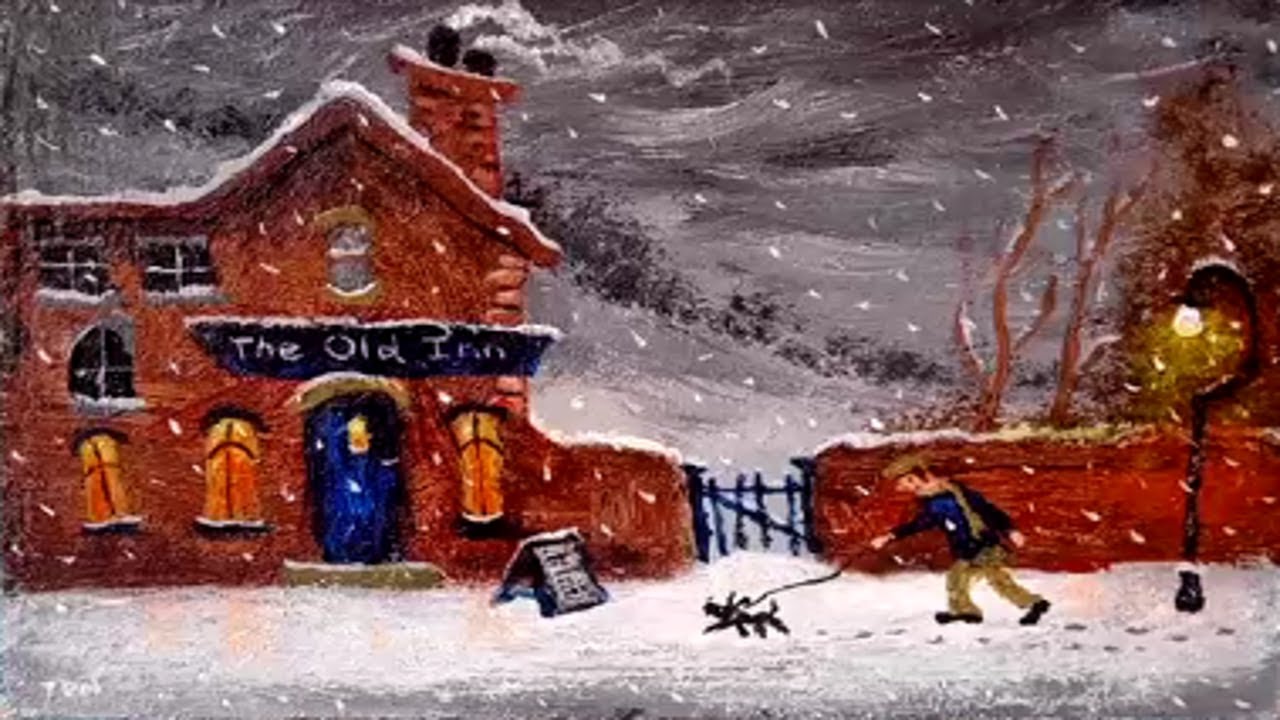This evocative illustrated image, reminiscent of a vintage postcard or Christmas card, depicts a snow-laden, blustery winter evening outside an inviting inn. The Old Inn, a brown brick building with a distinctive blue door and a black sign overhead emblazoned with "The Old Inn" in white lettering, stands warmly lit against the cold, grey surroundings. Golden light spills from three visible windows, suggesting a cozy refuge within, their glow contrasting with the dark, snowy sky. Smoke puffs gently from two chimneys atop the inn, adding to the scene's warmth.

In the foreground, a man bundled up in a jacket, scarf, and hat trudges through the snow, guided by his eager little black dog pulling at the leash. Footprints in the snow mark their path, hinting at others who have braved the storm. A black iron street lamp with a single, glowing lantern lights their way, while a sandwich board outside the inn hints at the offerings within. A fence with a gate encloses the inn's area, contributing to the scene's quaint charm, while snow-covered rooftops and swirling winter winds complete this idyllic seasonal tableau.